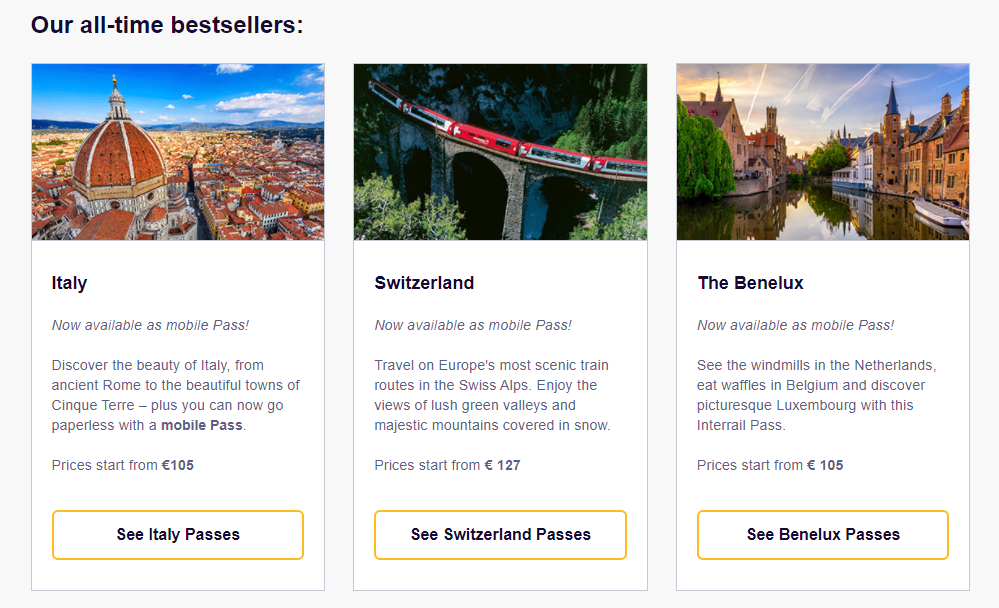This is a detailed descriptive caption for a travel site screenshot, highlighting advertisements for three popular destinations:

---

The screenshot showcases a travel site featuring advertisements for three top-selling destinations: Italy, Switzerland, and the Benelux. 

- **Italy**: The section for Italy is illustrated with a stunning photograph of a large, domed cathedral-like building overlooking the rooftops of the city beneath a bright blue sky. The accompanying text reads: "Italy now available as a mobile pass. Discover the beauty of Italy from ancient Rome to the charming towns of Cinque Terre. Plus, you can now go paperless with a mobile pass. Prices start from 105 euros."

- **Switzerland**: Switzerland's section features a captivating image of a long train traversing an arched bridge, surrounded by lush trees, seemingly journeying through the Swiss Alps. The text details: "Switzerland now available as a mobile pass. Travel on Europe's most scenic train routes in the Swiss Alps. Enjoy views of verdant valleys and majestic snow-capped mountains. Prices start at 127 euros."

- **Benelux**: The Benelux option presents a photo of quaint old brick buildings flanking a canal that winds through the scene under a bright blue sky. The description invites travelers: "The Benelux now available as a mobile pass. See the iconic windmills in the Netherlands, savor delicious waffles in Belgium, and explore picturesque Luxembourg with this interrail pass. Prices start at 105 euros."

---

Each section highlights the convenience of new mobile passes and the varying starting prices for these scenic and culturally rich travel experiences.